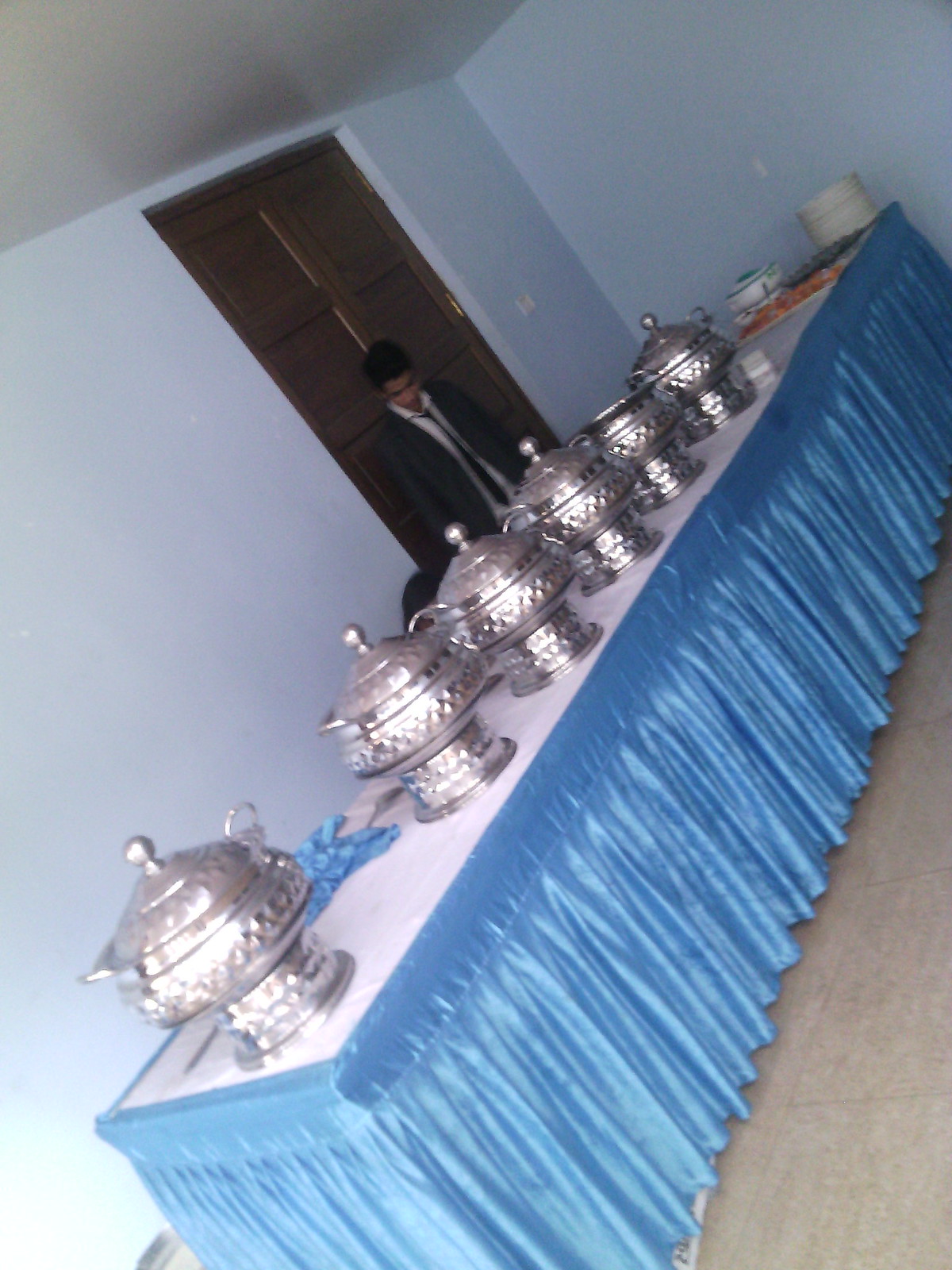The colour photograph, though tilted so that one needs to angle their head 45 degrees to the left for proper orientation, depicts a lavish banquet-style setup. The table, with its prominent long rectangular shape, is draped with a white tablecloth topped by a ruffled, light blue velvet-like skirt that extends nearly to the floor, effectively concealing the table's legs and any items beneath. The upper surface is adorned with six elaborate, embossed silver containers, reminiscent of urns, each crowned with rounded ball handles on their lids; notably, the fifth container is missing its lid. These containers are evenly spaced along the table. To the right, there are two flat platters of food, one dark and one red, accompanied by a white ceramic bowl. Additionally, a sizable stack of white plates is situated at the far right end. Behind the table, against a backdrop of light blue walls, stands a man dressed in a white shirt, tie, and black jacket; his dark hair is evident as he poses in front of a large brown wooden door. The banquet area is complemented by a beige tiled floor, creating a refined and formal atmosphere.